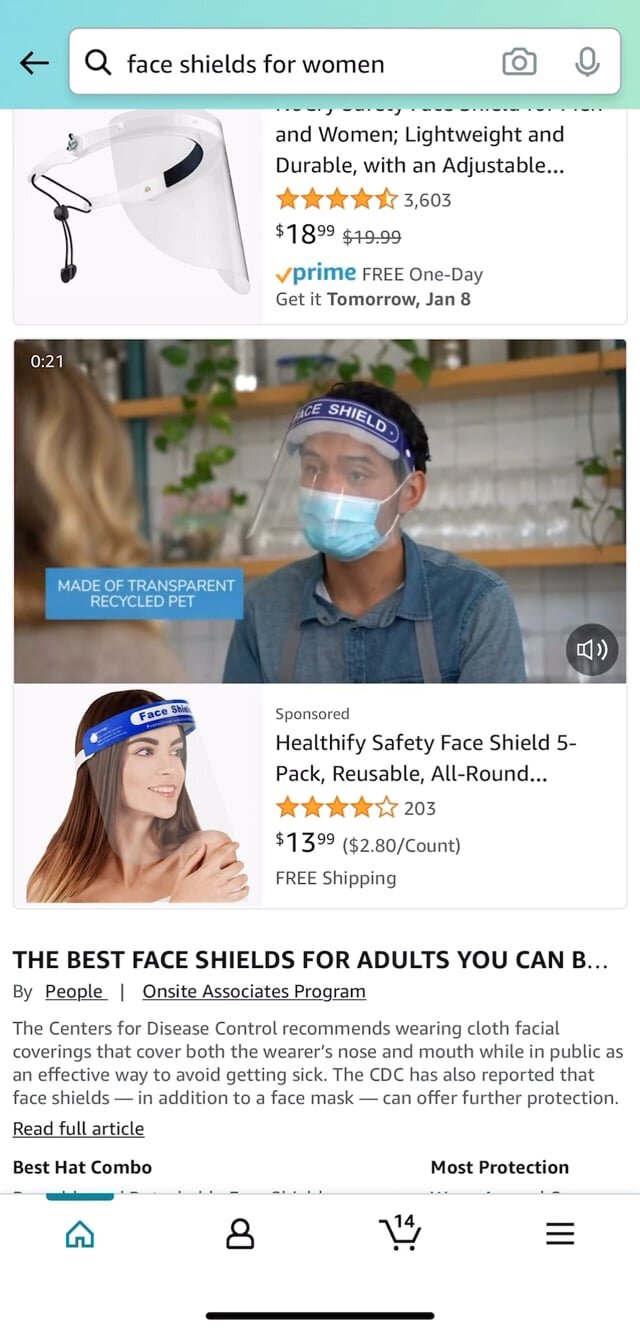This image is a screenshot from the Amazon shopping app featuring a search for "face shields for women." The upper portion displays a blue border with a white search bar where the search phrase "face shields for women" appears in black font. Below the search bar are search results showcasing various face shields.

The first product on the list, positioned to the left, boasts a high rating of around 4.5 stars. It is priced at $18.99, marked down from $19.99, with the original price crossed out. This listing includes the Amazon Prime logo in blue, accompanied by an orange checkmark, indicating "Free One-Day Delivery" with an estimated arrival date of January 8th. Additionally, there’s a 21-second video linked within this product display, featuring a man wearing the face shield. He is seen in a blue face mask and a bluish-gray shirt, standing in front of a backdrop filled with stacked wine glasses and a white-tiled wall. A woman with medium-length, light brown curly hair stands to his left.

Beneath this listing is a sponsored product featuring another face shield. The image shows a woman with long, straight brown hair and brown eyes, smiling as she models the shield. This second option is priced at $13.99 and has a rating of four orange stars. A snippet below this listing reads, "Best face shields for adults. You can be…" followed by truncated text, indicating additional details or a review further down.